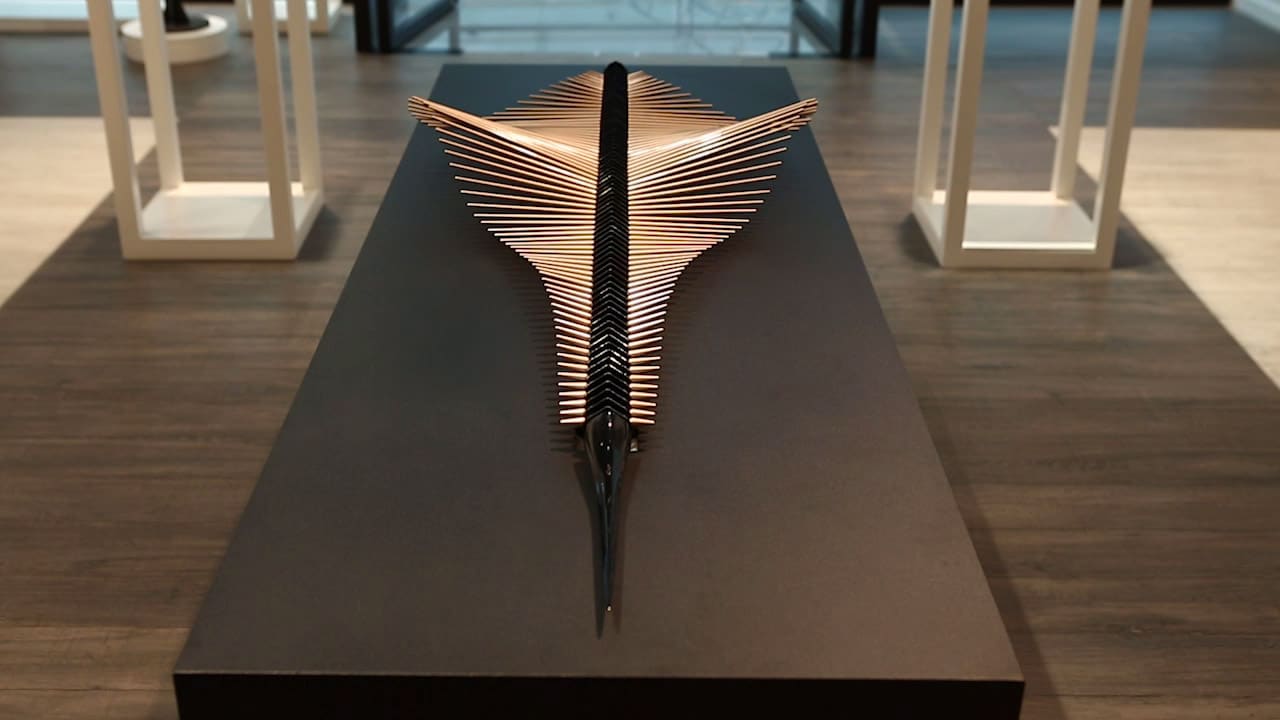In this indoor photograph, a striking piece of abstract artwork is prominently displayed on a large, dark grey rectangular platform placed on a brown wooden floor. The sculpture features a long black line at its center, flanked by numerous wavy, light brown wooden sticks of varying lengths, which create an undulating pattern reminiscent of a swimming fish. The floor also features white inverted stools, adding to the sense of an exhibit or modern art installation. The overall setting suggests a carefully curated artistic space, likely showcasing the intriguing and unusual nature of the central sculpture.